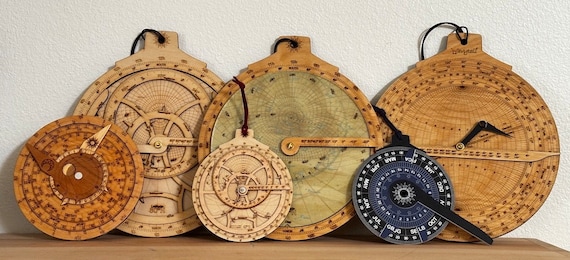The image depicts six intricately designed, round wooden ornaments arranged on a rectangular wooden surface with a textured cream-colored wall as a backdrop. The three larger ornaments are positioned in the back, while the three smaller ones lean against them in the front. Each ornament boasts a unique design resembling ancient navigational instruments such as compasses, astrolabes, or globes, complete with arrows, scales, and directional markings. Five of the ornaments are made of various shades of wood, ranging from light to dark tones, while one smaller ornament stands out with its blue color. All ornaments, except for one on the far left, have a black string threaded through a small hole at the top, suggesting they are meant to be hung. The detailed craftsmanship gives these ornaments an appearance of being handmade art pieces or decorative pendants.